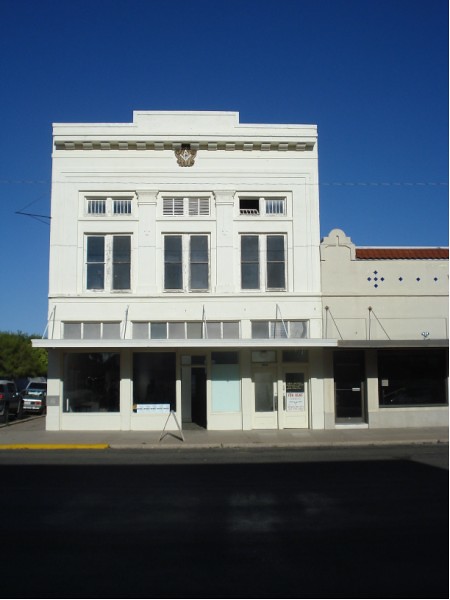This image depicts a two-story white stone building situated on the corner of a town square, viewed from across a dark-colored street with a visible sidewalk. The corner of the sidewalk has a yellow-painted curb. The building features an awning that stretches seamlessly from it to an adjacent one-story tan building on the right. The white building has three sets of windows with three transoms above them on the upper floor, and several signs in the windows on the first floor, though their content is indeterminate. Also notable are a small, unidentifiable sidewalk sign and a golden V-shaped symbol at the top of the building. The scene includes parked cars visible around the street corner and a clear blue sky in the background. Additionally, some power lines and trees are present to the left of the image, adding context to the setting.